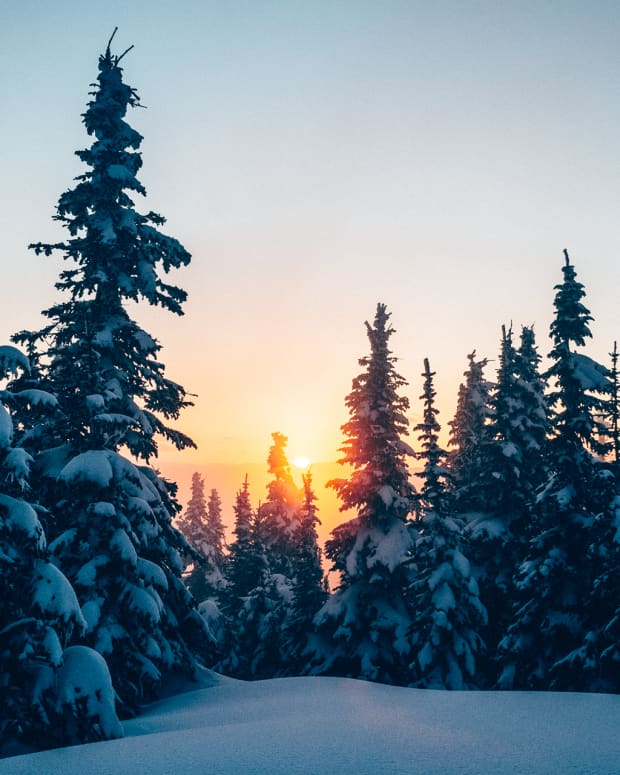In this serene winter scene, a cluster of 15 to 16 snow-covered evergreen trees, reminiscent of Christmas trees, stands majestically against a backdrop of a setting sun. The dark green needles of the trees are heavily laden with fluffy, tall mounds of snow, with occasional icicles hanging from the branches. The ground beneath them is also blanketed in a thick layer of snow. The sun, positioned in the middle of the photograph, casts brilliant yellow and orange hues that backlight the trees, highlighting some of them with a warm, golden glow. The sky above transitions from a neutral light gray to a soft blue, providing a tranquil setting for the nature scene. One particularly tall evergreen stands out among the others, its every branch adorned with snow, creating a picturesque winter landscape.